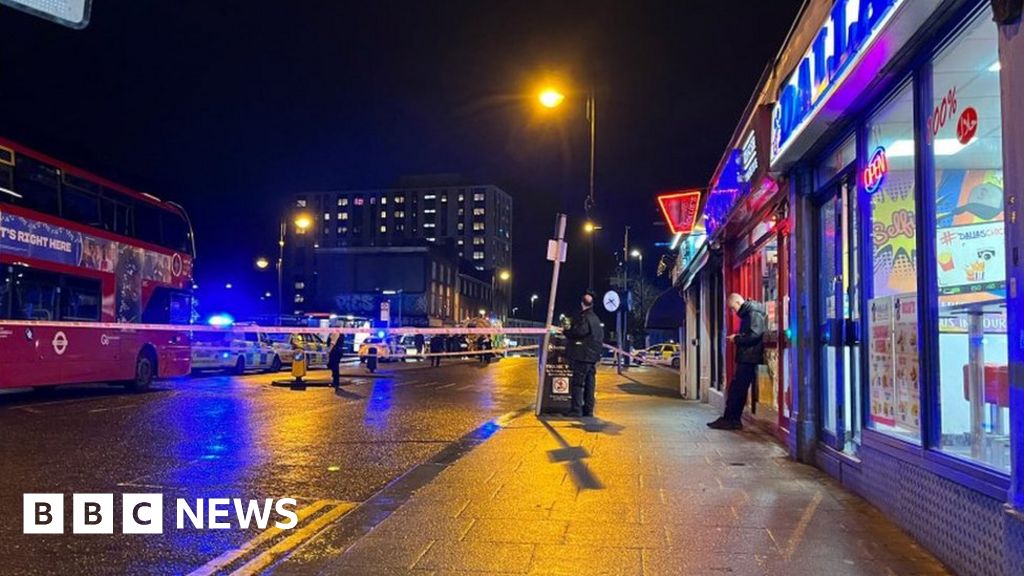The image captures a night scene on a clean, wet street in what appears to be London. The prominent features include a red double-decker bus stationed partially to the left. In front of the bus are police vehicles with flashing sirens and an area cordoned off with police tape, suggesting a potential crime or incident. The BBC News logo is displayed in white text on the lower left corner. On the right, a man engrossed in his phone stands in front of a brightly lit store, possibly a diner or a 7-Eleven, illuminated by LED lights. Another individual seems to be disposing of something nearby. The street is lined with various restaurants and kebab shops, and a yellow streetlamp casts a dim glow. In the distance, a multi-story tenement project housing unit looms, adding to the urban backdrop. The overall scene is dark, highlighted by the contrasting colors of the bus, streetlamp, and police lights.